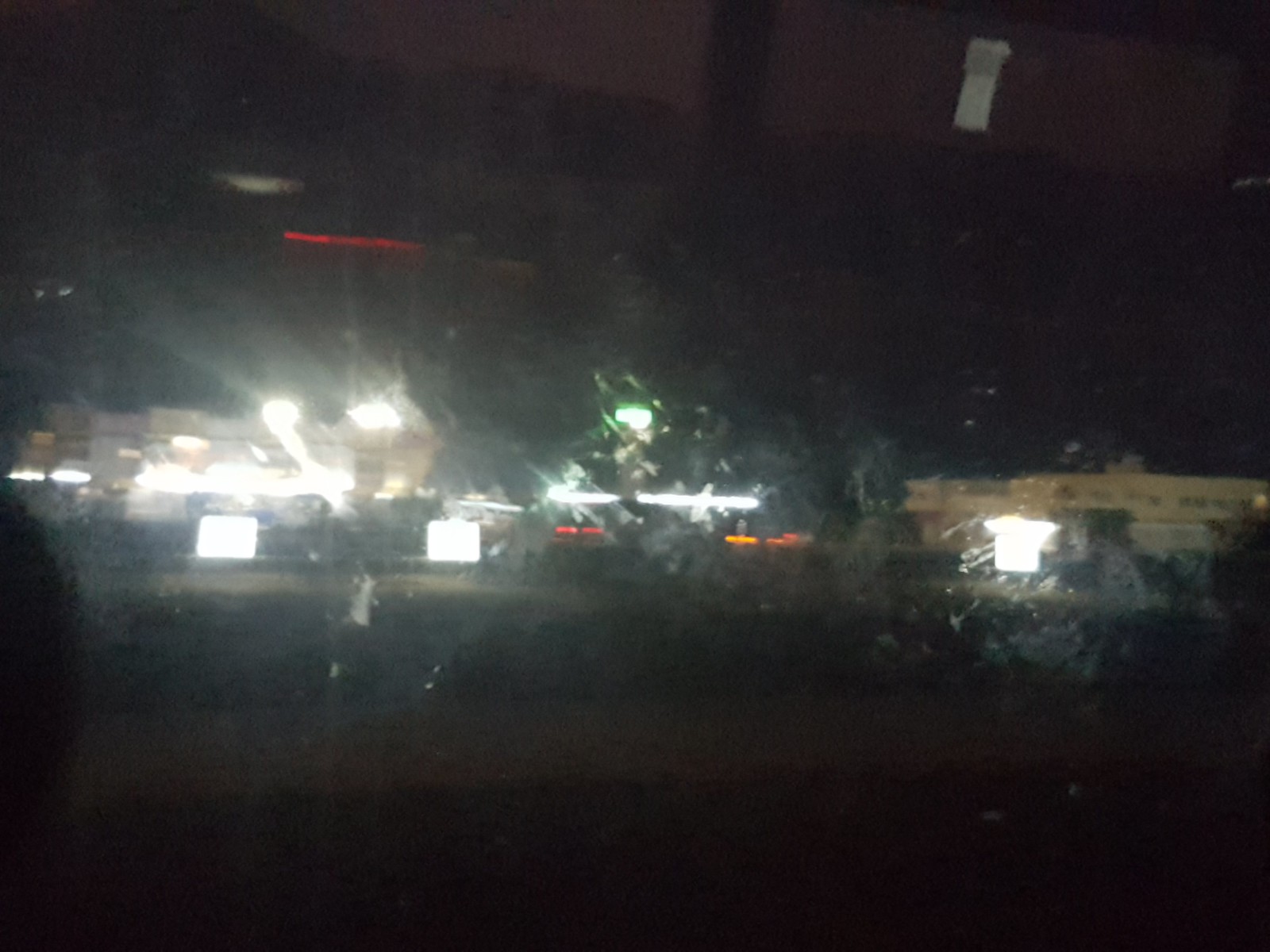The highly out-of-focus nighttime photograph captures a scene with numerous bright lights and reflections, likely exacerbated by taking the image through dirty or wet glass, possibly from inside a car. The bottom of the image features a black stripe, resembling a dark road, bordered by many white and colored lights, which appear to come from various sources. To the right, a structure that could be a gas station canopy is barely discernible, suggesting multiple gas stations might be within view, their floodlights blending together in the blurry distance. In the center, faint outlines of car lights can be seen, while to the left, brighter lights—potentially from a commercial building—dominate the area. The photo also includes a small red light streak in the sky and streaks of orange and red scattered throughout. The image is so grainy and indistinct that small details emerge sporadically, like the shadow of a head on the left side, and hints of a sidewalk with plants around a possibly small shopping center towards the background.